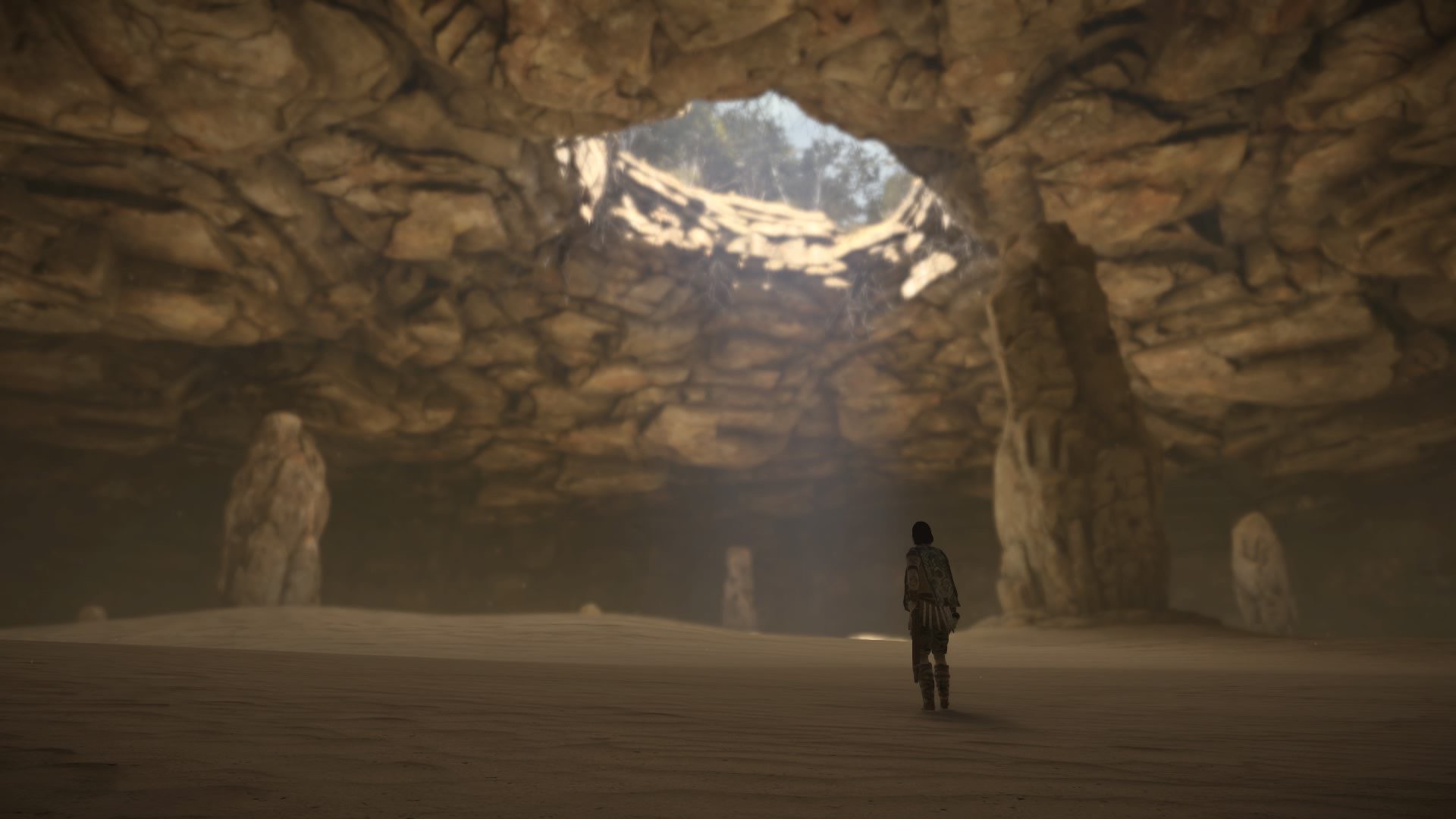A mesmerizing shot from a game or movie showcases a deep cavern illuminated by a shaft of sunlight piercing through a gaping hole in the rocky ceiling. Through the hole, blue sky and verdant treetops are visible, providing a stark contrast to the dark, sandy, and dirt-covered floor of the cave below. The cavern's ceiling is supported by at least four massive stone pillars that stretch from floor to ceiling, seemingly holding the structure together. In the lower right corner, a person clad in boots and a light-colored shirt strides purposefully toward the towering opening, their back turned to the camera. The scene exudes a sense of adventure and discovery, drawing the viewer into the mysterious underground world.